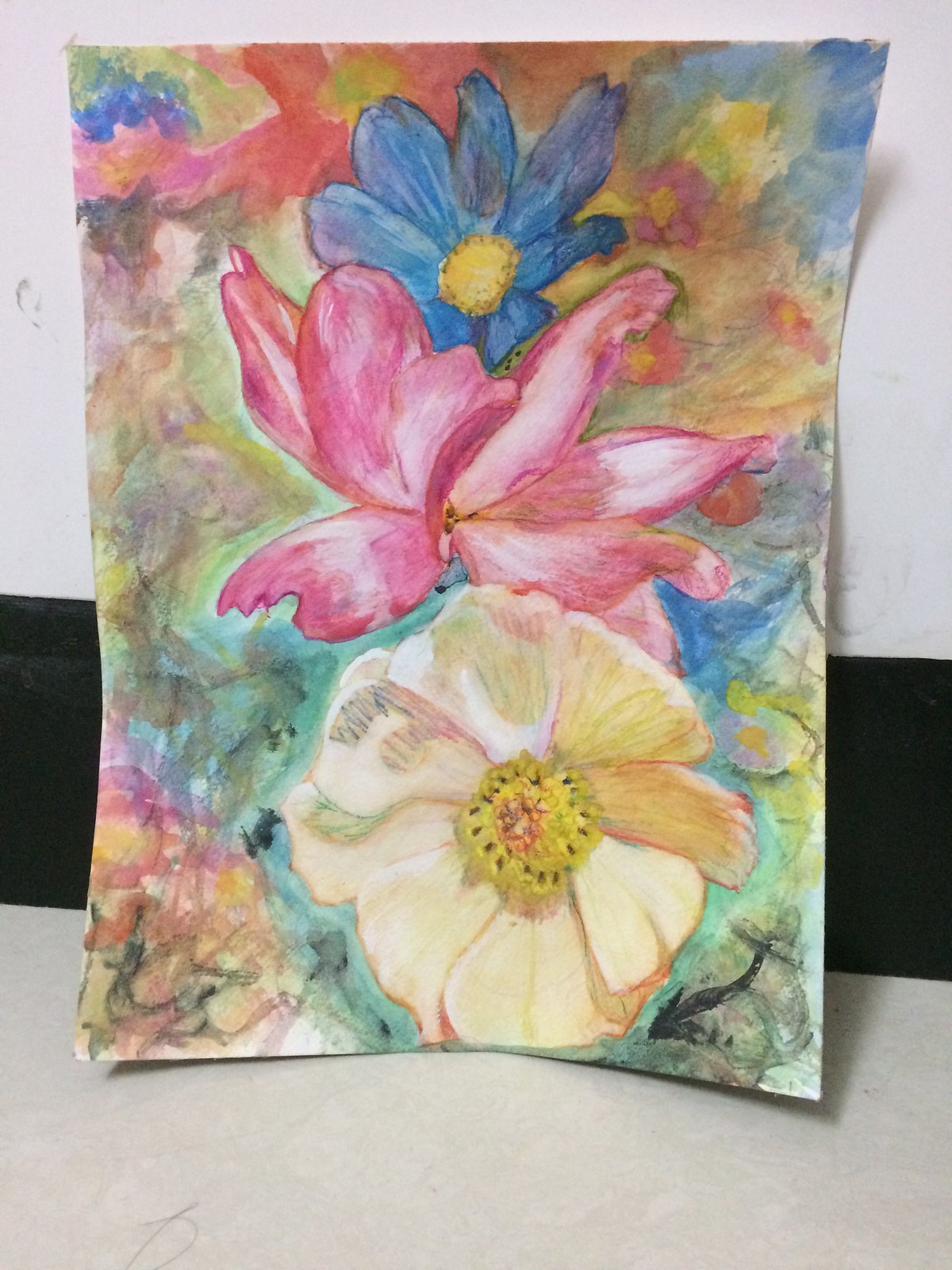This image showcases a handmade piece of art in portrait orientation, propped up against a wall where the upper portion of the wall is bright white and the bottom portion features a wide black trim. The artwork itself vividly captures three main flowers set against a vibrant and colorful background. At the top is a smaller blue flower with a yellow center, likely resembling a cosmos. Below it is a pink flower with elongated, flowing petals, and at the bottom sits a golden yellow flower with a darker center. The background is a harmonious blend of pink, red, blue, and green smudges, interspersed with hints of stems and distant floral shapes, creating a dynamic and colorful backdrop. The piece radiates artistic talent and appears to be crafted with watercolors, displaying the three prominent flowers in the center against the lush, blended background. The entire setup rests on what appears to be a lighter-colored counter or table, possibly gray or white.